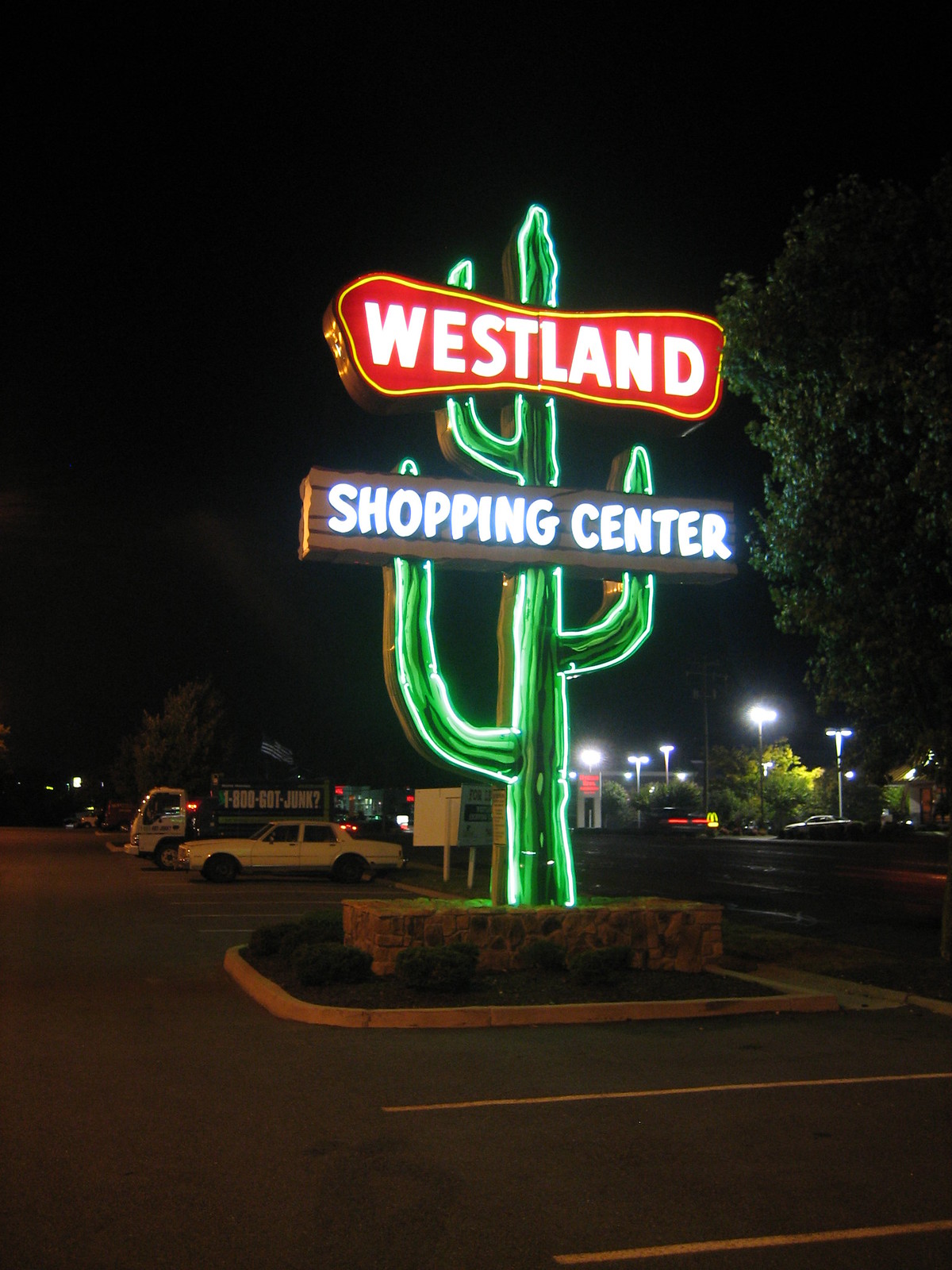The photograph, taken outdoors at night in a parking lot, captures a striking neon sign in the shape of a cactus, approximately 20 feet tall, prominently positioned on a stone base. The cactus sign features three arms and a long slender body, outlined in green neon lights with white highlights on the edges. At the top of the cactus, a red, irregularly shaped rectangle with a gold border displays the word "WESTLAND" in white neon letters. Below it, a rectangular wooden sign reads "SHOPPING CENTER" in white letters.

To the left side of the image, several cars and a truck are parked in designated spaces marked by yellow lines. The surrounding area includes a curb with small bushes, adding some greenery to the setting. On the right side, a road can be seen alongside a tree, with lights from a distant gas station illuminating the dark, starless sky. Street lights and parking lot lights provide additional illumination in the background. The atmosphere of the photo is clearly night-time, emphasizing the vibrant and eye-catching neon sign amidst the quieter surroundings.